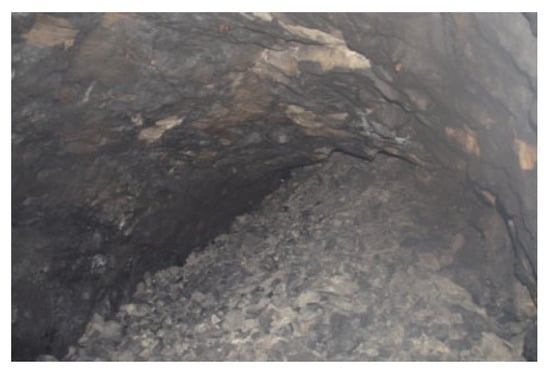This rectangular photograph, measuring roughly four inches wide by three inches high, captures a scene of a caved-in rock tunnel or pit, potentially resembling a cave, viewed from above. Dominating the scene is a large, arch-like formation of dark black-gray rock that spans from the lower left corner up to the top left and across to the upper right corner, then back down again. The archway, with its craggy texture interspersed with lighter gray and tan chips, hints at a natural or aged structural feature. Beneath this arch, starting just right of the center midline, a slope of small rocks and debris angles downward from the upper right towards the lower left, suggesting the aftermath of a landslide or rockslide. The rocky surface appears smoother on the left and more rugged on the right, with little white specks dotting the scene, possibly reflecting light. The image is somewhat blurred, especially in the upper right, where a bright area disrupts depth perception, making it challenging to discern the full extent of the cave-in. The overall color palette is dominated by shades of gray and black, with sprinklings of white and brown, enhancing the impression of this tunnel being old and collapsed.